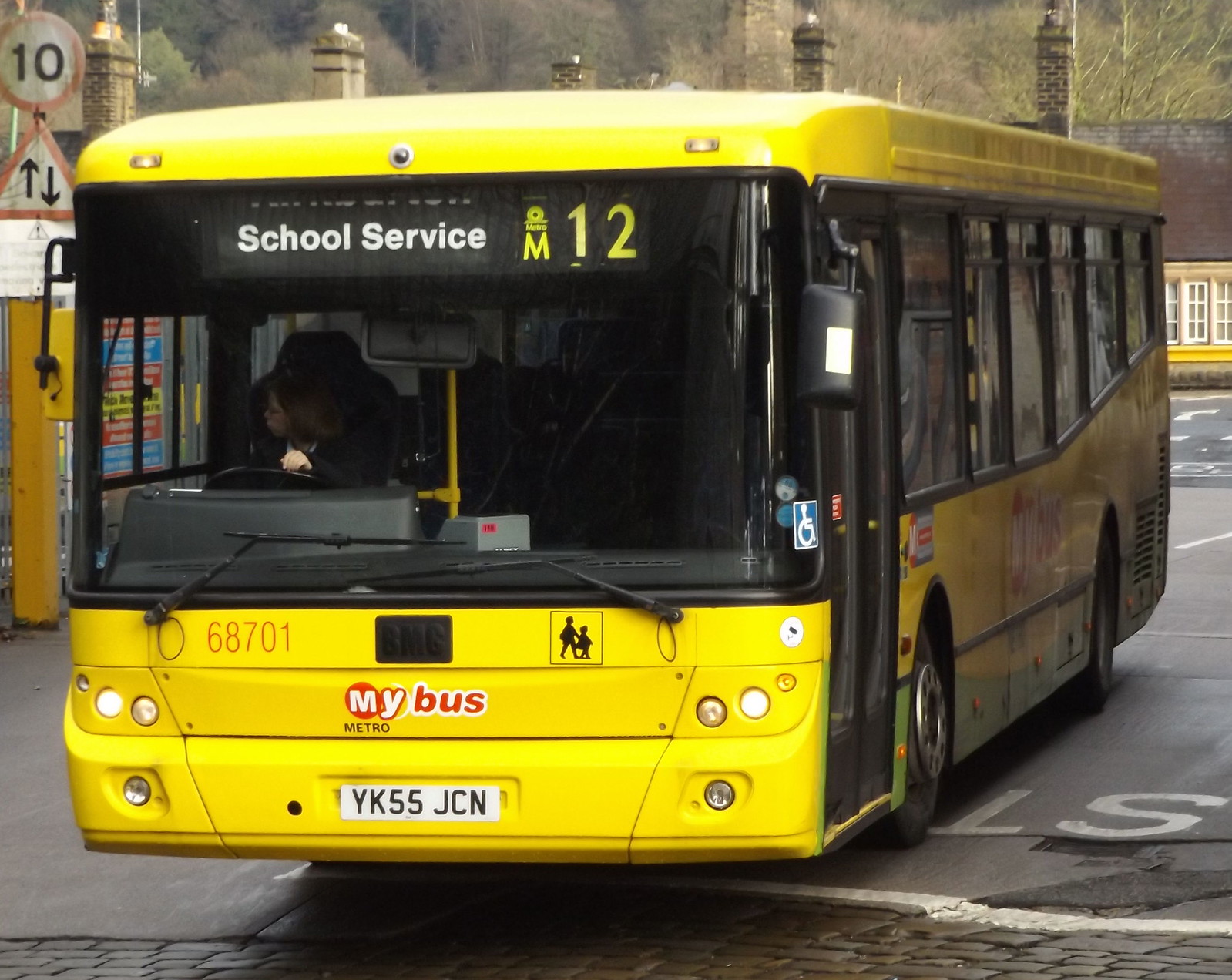The image captures a yellow school bus from "My Bus Metro" stopped at a stop sign while driving through the city. The bus, marked with the route number M12 and bus number 68701, displays the license plate YK55JCN. The female bus driver is visible through the windshield, looking to her right. In the background, there are buildings or houses with several chimneys and some trees. Additionally, on the left-hand side of the image, there is a street sign with the top part being a round sign indicating the number 10 and the bottom part being a triangular sign with an up and down arrow on it.